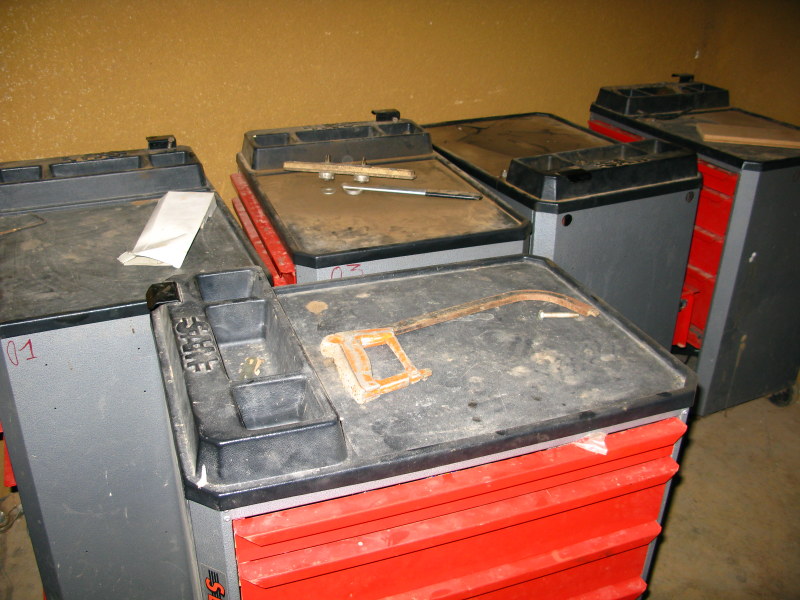This photograph depicts an old garage with five large tool cabinets lined up against a textured wall painted in an orange-brown or yellow-brown hue. The backdrop bears a slightly worn appearance, possibly resembling cardboard. The floor, which appears to be made of hard, painted concrete, shares a similar yellowish-brown tone. Each cabinet features distinct red drawers, silver sides, and black tops, all smeared with dust and debris, indicating a neglected state but also potential utility. The cabinets are topped with various small items, including a broken hand saw on the foremost cabinet and another unidentified tool towards the back. The cabinets are numbered in red paint, prominently displaying "01" and "03." Additionally, the top surfaces have small plastic compartments, ideal for organizing screws and other small implements. Overall, the scene suggests a once-functional workspace that now requires significant cleaning and organization.